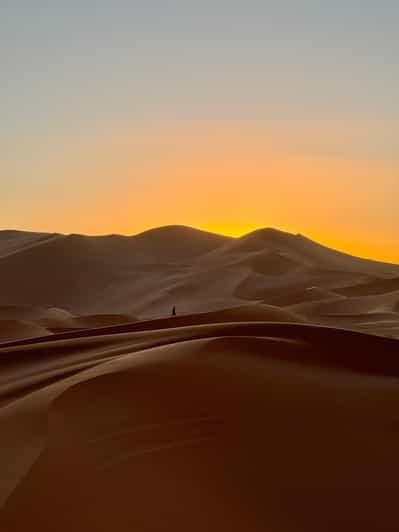In this image, a sprawling desert landscape showcases the mesmerizing beauty of sand dunes under a setting sun. The dunes, varying from caramel to dark, brown hues, display gentle slopes, pronounced curves, and waves across their surfaces, creating a dynamic and textured foreground. The sky above transitions from a deepening light purple at the top, through vibrant shades of peach and orange, culminating in a bright orange-yellow at the horizon where it kisses the sand dunes. Near the center of the image, a single figure, possibly dressed in black, walks towards the right. The smoothness of the sand closest to us is interrupted by two faint white-tan stripes, adding further contrast to the scene. As the eye moves up, the silhouette of the lone walker accentuates the tranquility and solitude of this picturesque desert at sunset.